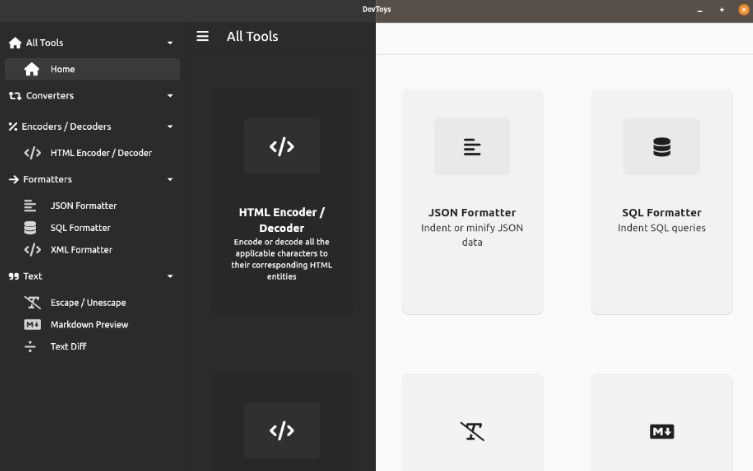This image features a comprehensive development tool interface. At the center of the screen, there is a section that details the available tools related to development activities. The left side of the interface has a black background, prominently listing a variety of utilities:

- Home
- Converters
- Encoders / Decoders
  - HTML Encoders / Decoders
- Formatters
  - JSON Formatter
  - SQL Formatter
  - XML Formatter
- Text Manipulation
  - Escape / Unescape
  - Markdown Preview
  - Text Diff

A specific tool's description is also provided: "HTML Encoder/Decoder - Encode or decode all the applicable characters to their corresponding HTML entities."

On the right side of the interface, set against a brown-tinted bar at the top, additional formatter tools are listed:

- JSON Formatter - Indent or minify JSON data.
- SQL Formatter - Indent SQL queries.

Below these descriptions, there's a boxed icon with a diagonal line crossing a text symbol, indicating a text suppression or removal feature. Another boxed icon is black with a white 'M' and a downward arrow, possibly representing a markdown download or action.

At the upper-right corner of the interface, there are standard window control buttons: an 'X' to close the interface, and '+' and '-' signs to maximize or minimize the window respectively.